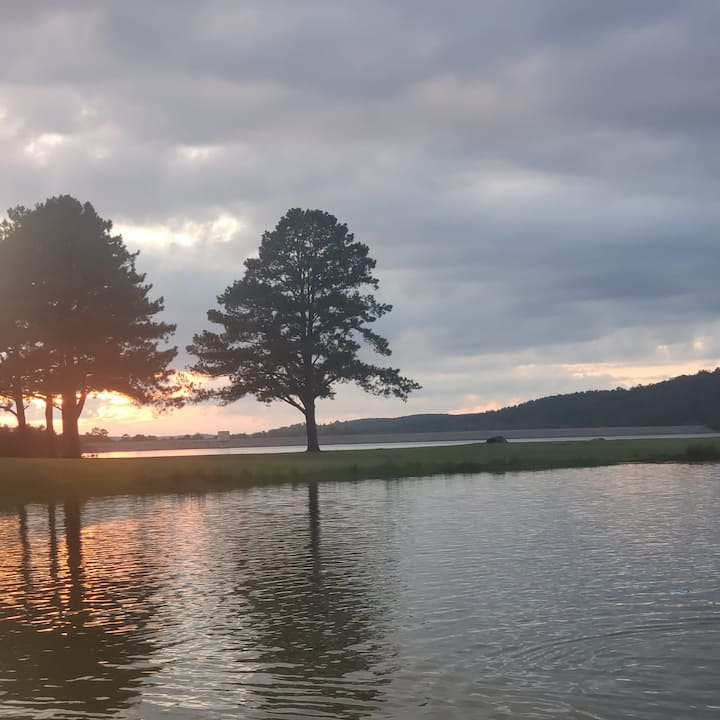The photograph captures a serene landscape at either sunrise or sunset under an overcast sky, creating a moody and tranquil atmosphere. Dominating the center of the image is a narrow peninsula, or maybe an island, that separates two sections of the lake. This strip of land is adorned with two prominent deciduous trees, one slightly to the left and the other to the right, along with several other trees in the background. The trees are fully grown with dark-colored leaves, and their reflections cast softly on the surface of the lake, emphasizing the stillness of the water.

The sky is filled with thick gray clouds, allowing only a few patches of light to seep through, revealing hints of pale white and pink hues—a gentle touch of the concealed sun. In the background, rolling dark gray hills or mountains add a sense of depth and enclosure to the tranquil scene. The foreground features a notably calm lake, reflecting both the muted colors of the sunrise or sunset and the silhouettes of the trees, enhancing the overall peaceful and slightly melancholic tone of the photograph.